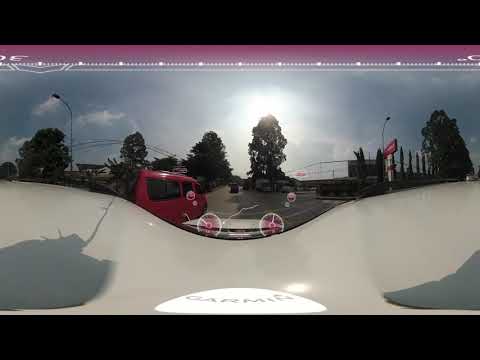This image is a colored outdoor photograph that appears to be taken from behind a screen, resembling a computer display or a photo encased in cellophane, with black borders on the top and bottom framing it. The top edge features a pinkish bar with a texture reminiscent of a Ziploc bag, dotted with white, creating a line across it. The scene within the photo seems to be a warped, panoramic view, distorting the elements into a curving, almost surreal representation.

At the heart of the image is a warped street scene featuring a squished red van on the left, flanked by tall trees on either side. The trees, which likely have green leaves, appear dark due to the sunlight casting strong shadows. A gray-colored street stretches out, accompanied by a large gray building on the right, identifiable by its white wall. There are also a few lampposts and a white and red sign in the scene.

The sky is a mix of bluish-gray hues, providing a slightly gloomy ambiance, punctuated by white clouds. Curiously, in the center of the image, a bright white ring of light, potentially the sun, draws attention. Near the bottom center, the word "Garmin" is evident on what looks like a white, almost pyramid-shaped object caught in the distortion. Additionally, there are reflections, including two white and red wheels, contributing to the unusual composition. The photograph’s overall effect is surreal, as if viewed through a curvilinear lens or a windshield.